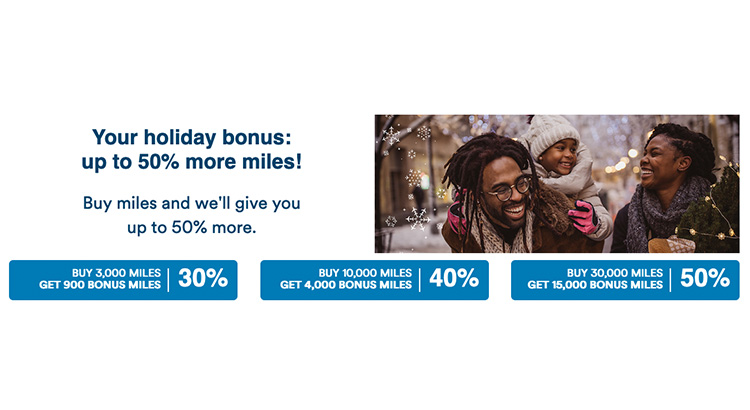**Holiday Bonus Promotion Advertisement**

The advertisement promotes a special holiday bonus offer with up to 50% more miles for customers purchasing miles. The details of the promotion are as follows: 

- Buy 9,000 miles and receive 900 bonus miles, a 10% bonus.
- Buy 10,000 miles and receive 4,000 bonus miles, a 40% bonus.
- Buy 30,000 miles and receive 15,000 bonus miles, a 50% bonus.

On the right side of the ad, there's a heartwarming image of a family enjoying a festive moment outdoors, adding warmth and an inviting touch. The dad carries a child on his back, and the mom smiles at them, encapsulating the joy of the holiday season. The background features snowflakes and holiday lights, enhancing the seasonal feel of the advertisement.

The ad predominantly uses white and blue colors, creating a clean and straightforward design. Despite the wintry themes, the family's attire suggests a milder climate, indicating the use of stock photography.

Overall, the ad successfully conveys the holiday spirit and effectively communicates the attractive bonus offer.